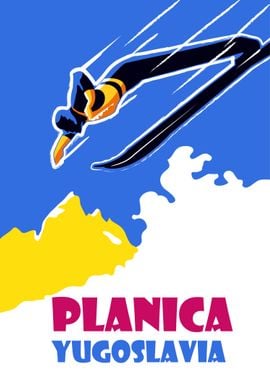This vibrant and stylized poster features a highly abstract depiction of a downhill skier racing down a mountainside. The poster uses a palette of medium blue, rose pink, yellow, and black. The skier, dressed in a black athletic ski outfit with a yellow bib and black helmet, is positioned in the upper right corner, leaning dramatically forward over their long black skis, suggesting high velocity with white motion lines trailing behind. They descend diagonally from the upper right to the lower left center against a background of a bright blue sky. Lower in the composition, a snowy white mountain peaks up at a slope beneath the skier, with a prominent yellow mountain, possibly depicting the Matterhorn, occupying the left middle section of the poster. At the bottom, large dark pink text reads "PLANICA," with "YUGOSLAVIA" in a slightly smaller, dark blue font below it. The overall design is dynamic and eye-catching, emphasizing speed and motion in a simplistic yet striking manner.